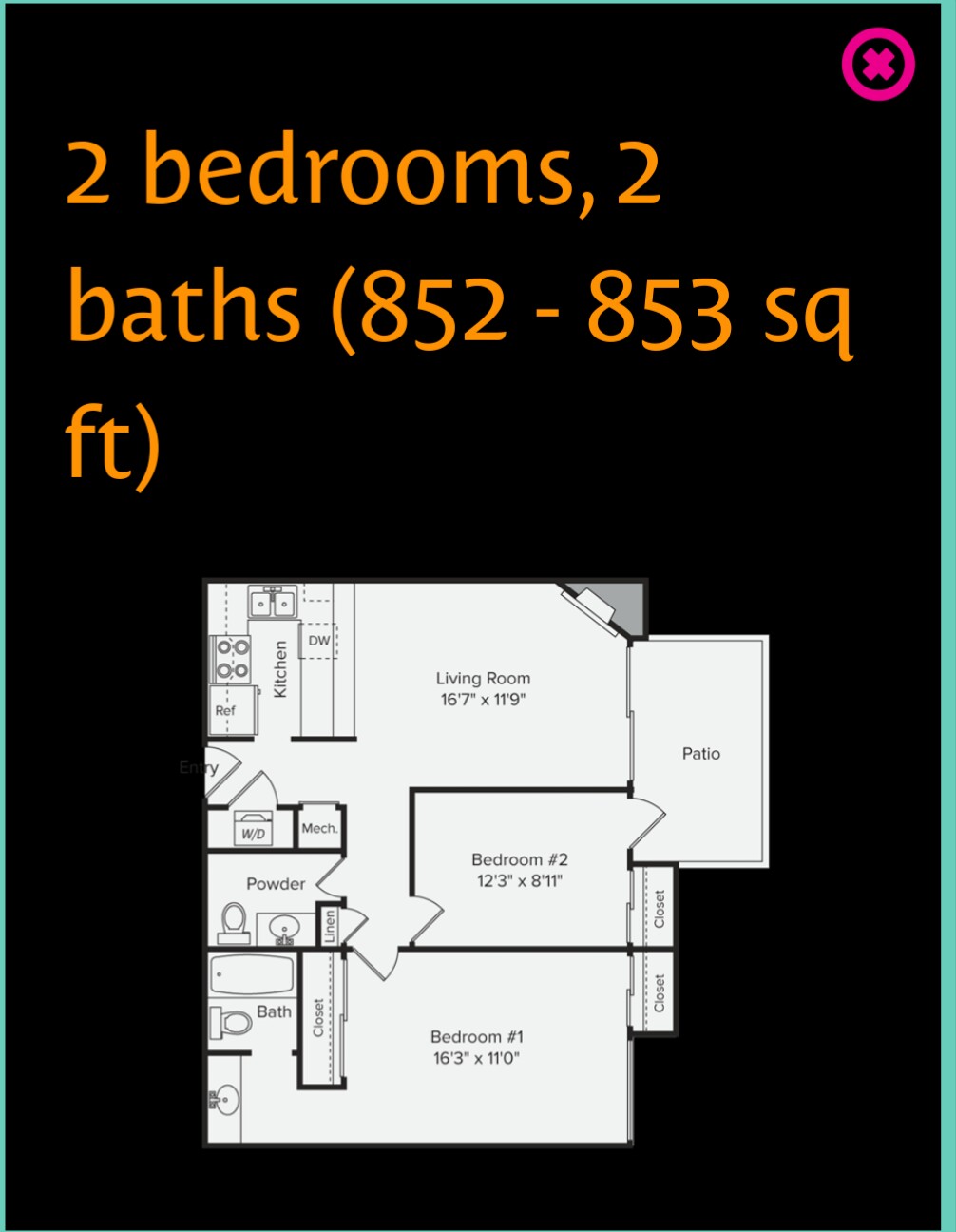The listing features a detailed floor plan for an 852-853 square foot apartment, highlighted in orange text on a black background. The layout showcases two bedrooms and two bathrooms, with additional room dimensions provided. A prominent pink 'X' within a circle marks a specific area in the upper right corner of the map. 

The floor plan includes:
- A larger primary bedroom with two closets and an en-suite bathroom.
- A second, smaller bedroom with a single closet.
- A hallway-separated powder room accessible from the second bedroom.
- A compact kitchen equipped with a stove on one side and a double sink centered at the back.
- A living room and a patio for added living space.

This detailed, easy-to-navigate floor plan offers prospective tenants a clear visualization of the apartment's layout and amenities.